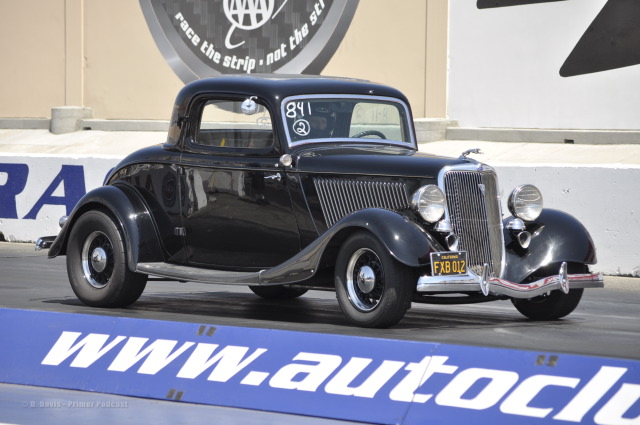The photograph depicts a classic black coupe, likely from the 1930s or 1940s, situated on what appears to be a racing track or speedway. The car features smoothly flowing lines typical of that era, with a prominent chrome front grille and large headlights. The front grille bears a logo that resembles the Jaguar emblem. The coupe has modified wheels, with the rear wheels being notably wider than the front. The license plate reads FXB 0112, and to the left of the bumper, there's a hint of a chrome color. Written on the windshield in white paint are the numbers "841" with a circled "2" beneath them. 

Inside the car, you can see a driver wearing a black helmet, positioned near the steering wheel. In the foreground of the image, there is a blue sign on the ground displaying a partially visible URL, www.autoclub or www.autotalk.com, with the latter part cropped out. To the left of the image, a white wall features advertising text in dark blue, partially visible with only the letter "A" legible. Additionally, there is a larger wall in the background, transitioning from cream to white, adorned with a black and silver circular logo containing the letters "AAA". A slogan reading "erase the strip not the strip" is partially discernible above a semicircular silver element near the blue sign. Overall, the image captures the essence of a vintage racing scene, highlighting the elegant yet powerful design of the old-school coupe.